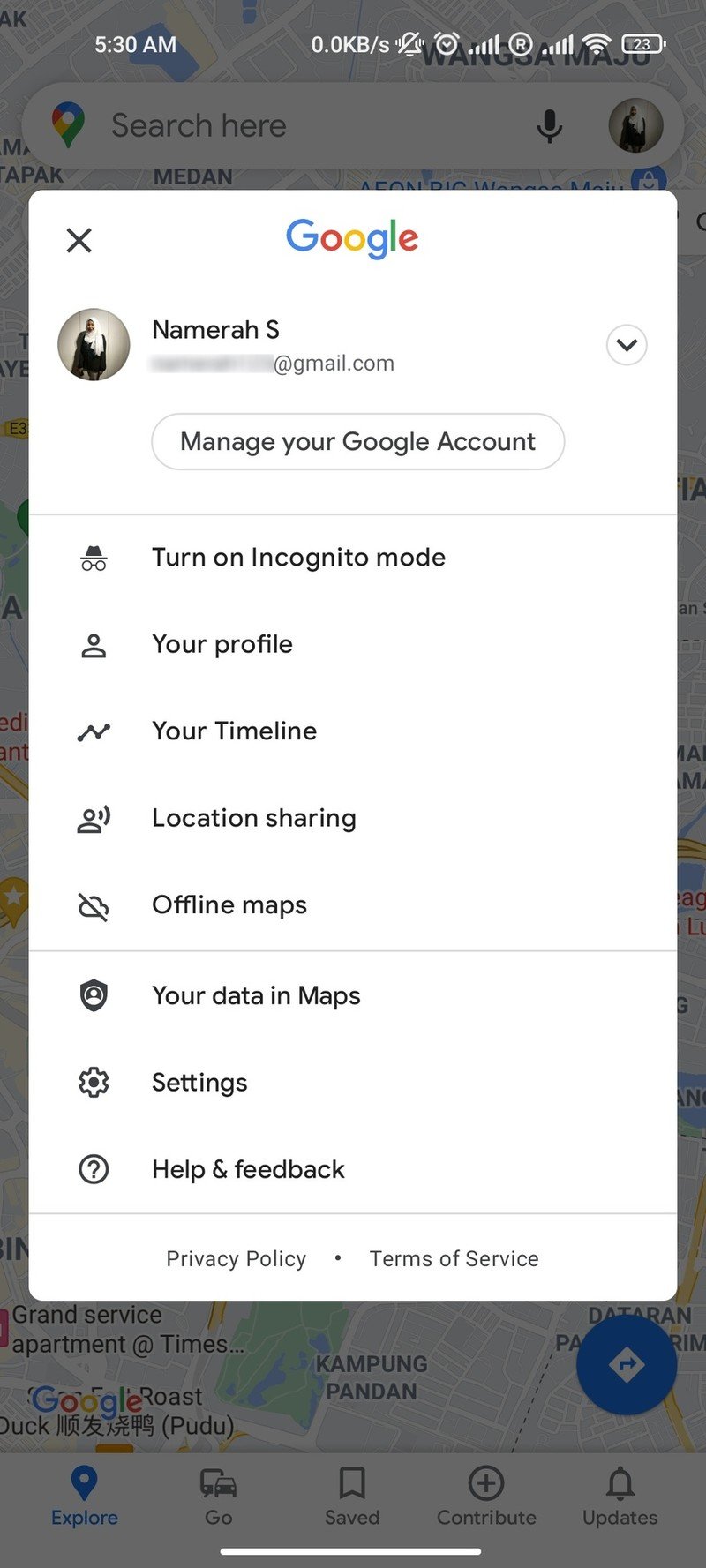A detailed caption for the given image could be:

---

A screenshot of a Google Maps interface on a cell phone taken at 5:30 a.m. The screen exhibits a subdued grey tint, typical of a night mode or dark theme. The map, showcasing an area somewhere in India, is somewhat obscured due to the grey filter, making it harder to discern specific locations. At the top of the screen, a search bar is visible, containing a push pin icon and a microphone icon for easier access. To the right of the search bar are additional interface icons. A pop-up window is prominently displayed, featuring an 'X' in the top left corner to close the window, a Google icon at the center top, and the title "From Nomera S." beneath it, with the email partially blurred out to maintain privacy. Below the email, there's a blue button labeled "Manage your Google Account." The window also displays several options including "Turn on Incognito mode," "Your profile," "Your timeline," "Location sharing," "Offline maps," "Your data in Maps," "Settings," and finally, "Help and feedback."

---